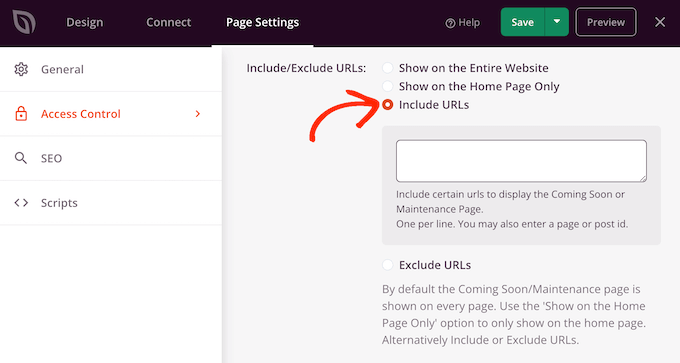The interface depicted in the image features a grey background with various sections and settings for a webpage. The top menu includes tabs labeled "Design," "Connect," and "Page Settings," with "General," "Access," "Control," and "Scripts" displayed in white text. 

On the right side, there is a 'Help' icon, represented by a circle enclosing a question mark. Below that, a red button labeled "Save" is situated next to a green rectangle containing the "Preview" option. Additionally, there is a feature labeled "Exclude URLs."

The image further includes three radio buttons with the following options: "Show on the entire website," "Show on the homepage only" (highlighted in red), and another unnamed option. An arrow, also in red, points directly at the "Show on the homepage only" radio button.

Below these settings, a white text box provides space to "Include certain URLs to display the coming soon or maintenance page, one per line." There is also an option to enter a page or post ID to exclude URLs. Instructions clarify that, by default, the coming soon or maintenance page will display on every page, unless the "Show on the homepage only" option is selected. Alternatively, users have the option to include or exclude specific URLs.